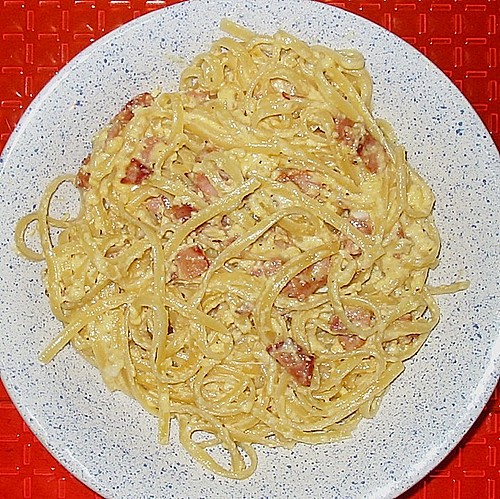This top-down image showcases a large serving of pasta, likely linguine or flat ribbon noodles, bathed in a rich, cream-based carbonara sauce. The pasta is generously mixed with small pieces of bacon, contributing to its hearty appearance. The dish sits atop a distinctive white plate adorned with dark blue speckles, which is nearly filled with the saucy pasta. This white, speckled plate contrasts vividly with the red, metallic-looking background featuring a square pattern. The absence of utensils or text further draws attention exclusively to the inviting, well-sauced pasta dish in the center of the composition.